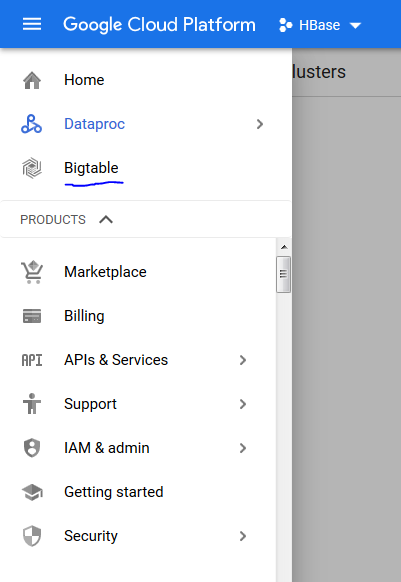The image displays a detailed view of the Google Cloud Platform (GCP) user interface. On the left side of the screen, the three horizontal lines (often referred to as the "hamburger menu") are clicked open, revealing a comprehensive navigation panel. This expanded menu lists multiple options, starting with 'Home,' followed by 'DataProc' which is highlighted in blue, indicating it is currently selected. Next, there is 'Bigtable,' underlined in blue, suggesting it is a sub-category or secondary selection under the highlighted option.

Below these primary options, the menu expands to show other main categories like 'Products,' 'Marketplace,' 'Billing,' 'APIs & Services,' each accompanied by a right-facing arrow, indicating that further sub-options are available upon selection. Other notable sections include 'Support,' 'IAM & Admin,' 'Getting Started,' and 'Security,' all of which also feature the right-facing arrows for additional configuration or information options.

An HBase option is visible with a down arrow, suggesting it has a dropdown menu for more selections. Overall, this image captures the robust and hierarchical structure of the GCP navigation menu, emphasizing the platform's depth of options and user-targeted configurations.